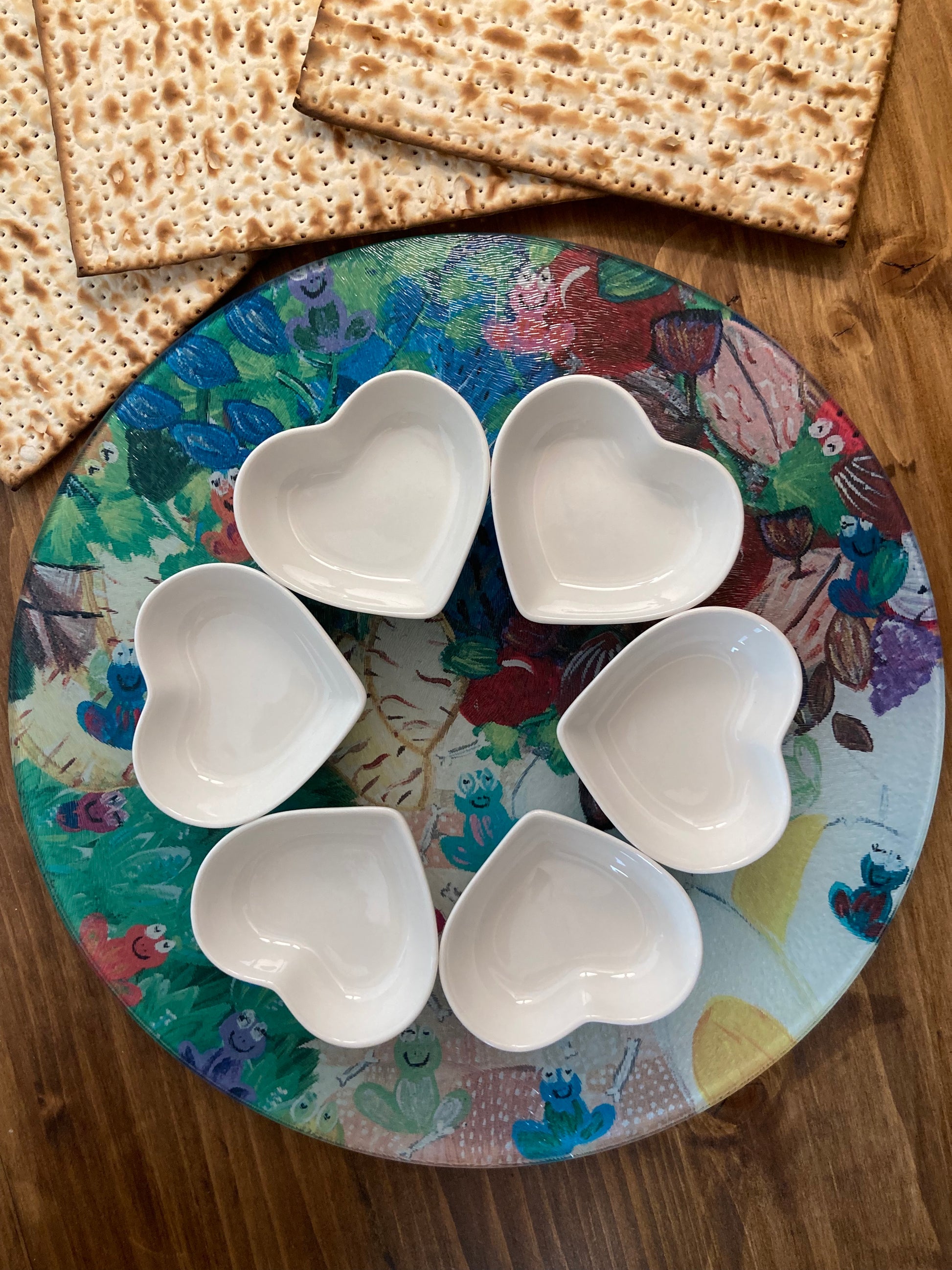In this overhead image, a beautifully detailed spread is showcased on a rich brown wooden table. At the center is a vibrant, colorful dish adorned with an eclectic mix of intricate designs featuring small blue and green bugs, whimsical frogs, and an assortment of flowers and fruits, including distinctly visible grapes on the right side and a blue frog on the lower right. Nestled within the dish are six pristine white heart-shaped bowls, all empty and arranged neatly. In the upper left corner of the image, three golden-brown matzah crackers are partially visible, fanned out like a deck of cards. The matzahs display characteristic rows of tiny perforations and exhibit a slightly darker toasting along their edges, adding a touch of rustic charm to the scene.